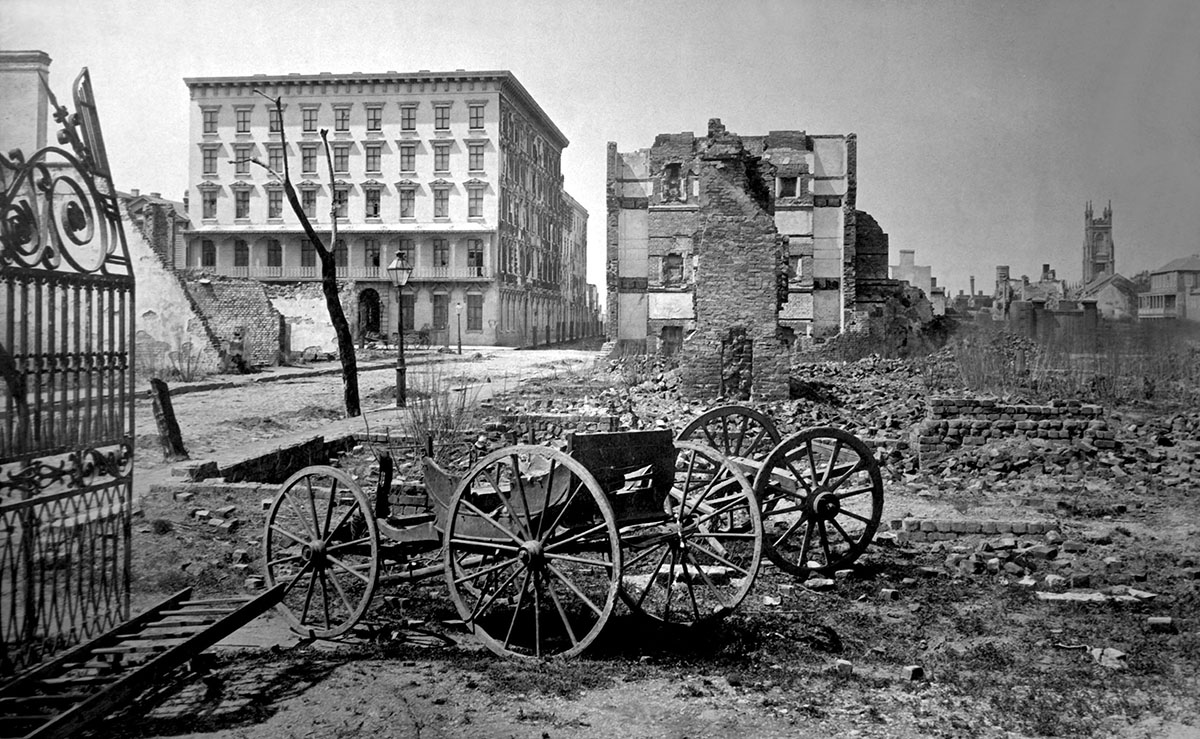The black-and-white photograph depicts a desolate, war-torn scene, possibly dating back to the 1920s or 1930s. In the foreground, amidst a sea of rubble and broken brick, lie the remnants of what were once two horse-drawn carriages, identifiable by their large wooden wheels. Nearby, a crumbling brick fireplace stands as a lone sentinel amidst the ruins, suggesting that a building once stood here but has now mostly collapsed. An old-fashioned street lamp rises from the debris, casting an eerie shadow over the decimated landscape. To the left, a large iron gate stands ajar, hinting at what was once a demarcated area now lost to destruction. The background reveals further devastation: one building, though partially intact with several floors and windows, contrasts sharply with its neighbor—a severely damaged structure missing its top layer. Barren trees line an old dirt roadway, accompanied by vintage light posts, completing the image of a city ravaged by conflict long ago.